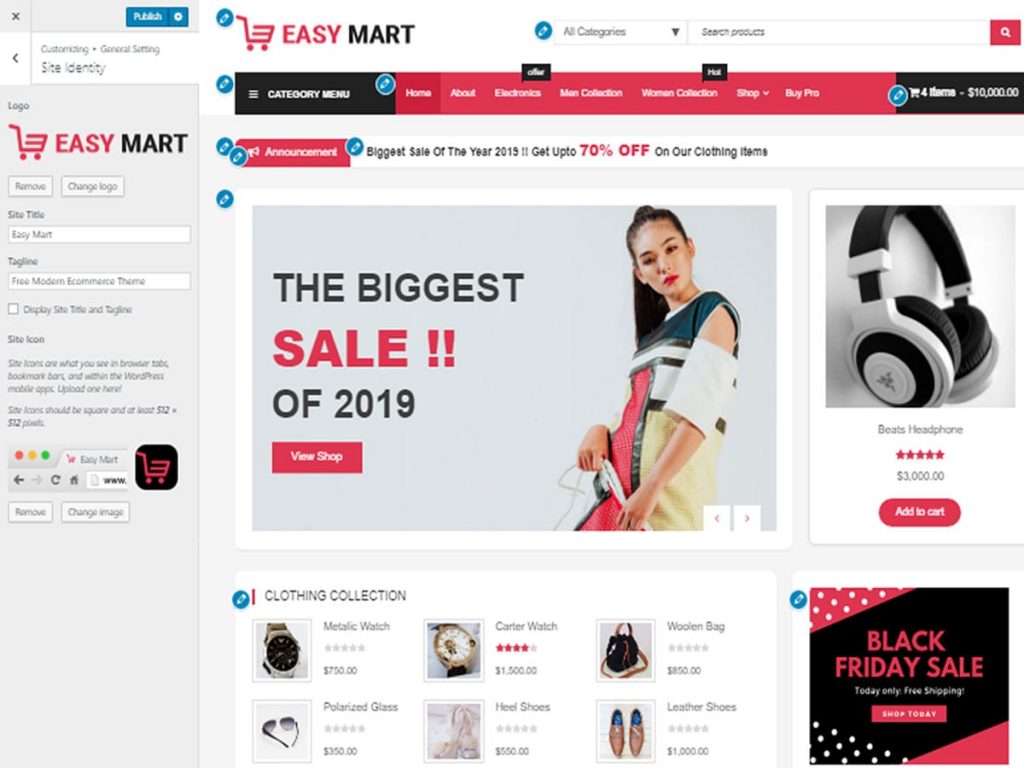This image is a screenshot of the Easy Mart online shopping website displayed on a laptop. On the left side of the page, the Easy Mart logo and the site’s name are prominently featured, along with a small grocery cart icon. Towards the top, there is a search bar allowing users to type in specific items they want to find, next to an 'X' icon. 

The right side of the page has a navigation bar running across the top with various categories including Home, About, Electronics, Men's Collection, Women's Collection, Shop, Buy, and Pro Buy PRG. Below this, there is a section resembling a grocery checkout page and several advertisements.

One of the ads towards the top depicts a girl with a ponytail looking at the screen, accompanied by the text "The biggest sale of 2019, View Shop". Below this, near the bottom of the page, a banner reads "Black Friday Sale". In the upper right section of the page, there is an advertisement for Beats Headphones priced at $3,000, with a five-star rating. 

The bottom left section of the page showcases a variety of products including watches and a pair of shoes, providing images, descriptions, and prices for six items in total.